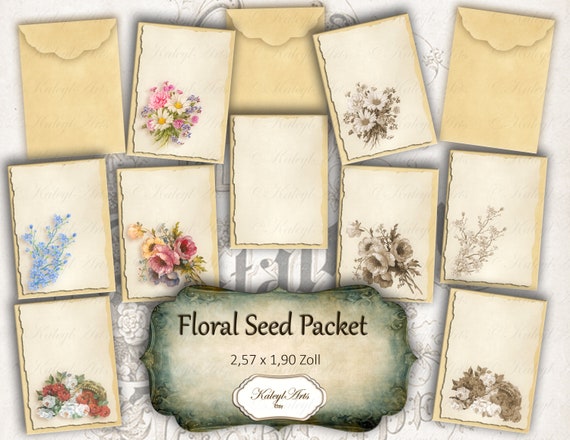The image depicts a series of floral seed packets, meticulously arranged against a white background. At the bottom of the image, text in black font reads "Floral Seed Packet" alongside the dimensions "2,57 x 1,90 ZOLL." The packets, varying in color from light brown to beige, feature an assortment of floral designs. These designs are an eclectic mix of colors including white, pink, purple, blue, orange, and brown. Some of the flowers are depicted in vibrant hues, while others have a vintage sepia tone, lending an antique feel to the collection. Scattered among the vivid illustrations, a few envelopes of a slightly darker shade than the notecards are visible. One notecard in the center stands out as it remains blank, providing a stark contrast to the surrounding florals. An elegant cursive script is present at the bottom, though not entirely legible, adding a touch of sophistication to the overall composition.